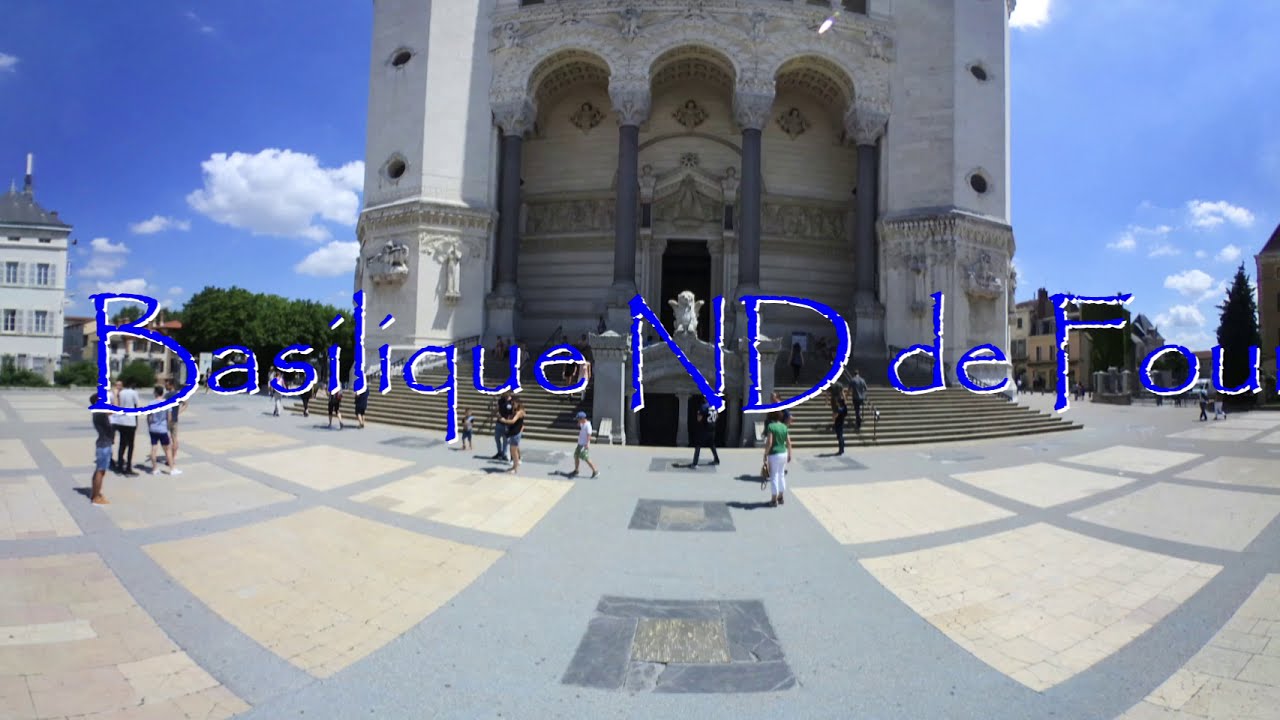This panoramic image captures a bustling city square, featuring the iconic and ornate entrance of the Basilica of Notre Dame. Dominating the center of the image is bold, blue text, reading "Basilique N-D-F-O-U." In front of the grand, light-colored cathedral-like structure, whose façade is adorned with intricate arches and four light gray columns, lies a checkerboard courtyard made of light blue and white bricks. People mill about, some taking pictures, while others ascend the numerous steps leading to the entrance, which includes a sub-entrance and small statues of notable figures above the doorway. Flanking the scene are pieces of nearby buildings, one to the left, which is two or three stories high, and another on the far right. The sky above is partly cloudy, and trees frame both sides of the courtyard, enhancing the picturesque and historical ambiance of this landmark area.